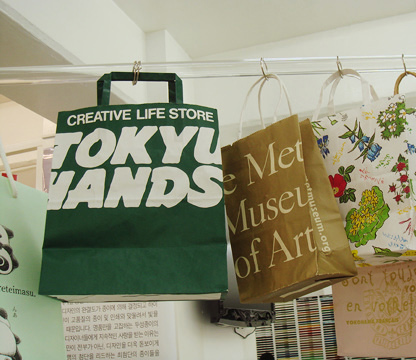The image depicts a square photograph taken inside a room or store with white walls and ceiling. A clear horizontal pole is used as a rack to hang a variety of bags. In the center, there is a green paper bag with white text partially visible, stating "Creative Life Store, Tokyu Hands." To its right, a brown bag features the words "The Met Museum of Art." Further to the right, there is a white bag adorned with colorful flowers. The background includes a stack of items at the bottom, possibly CDs or other stored materials, and a leaning sign with numerous symbols in a non-English language.